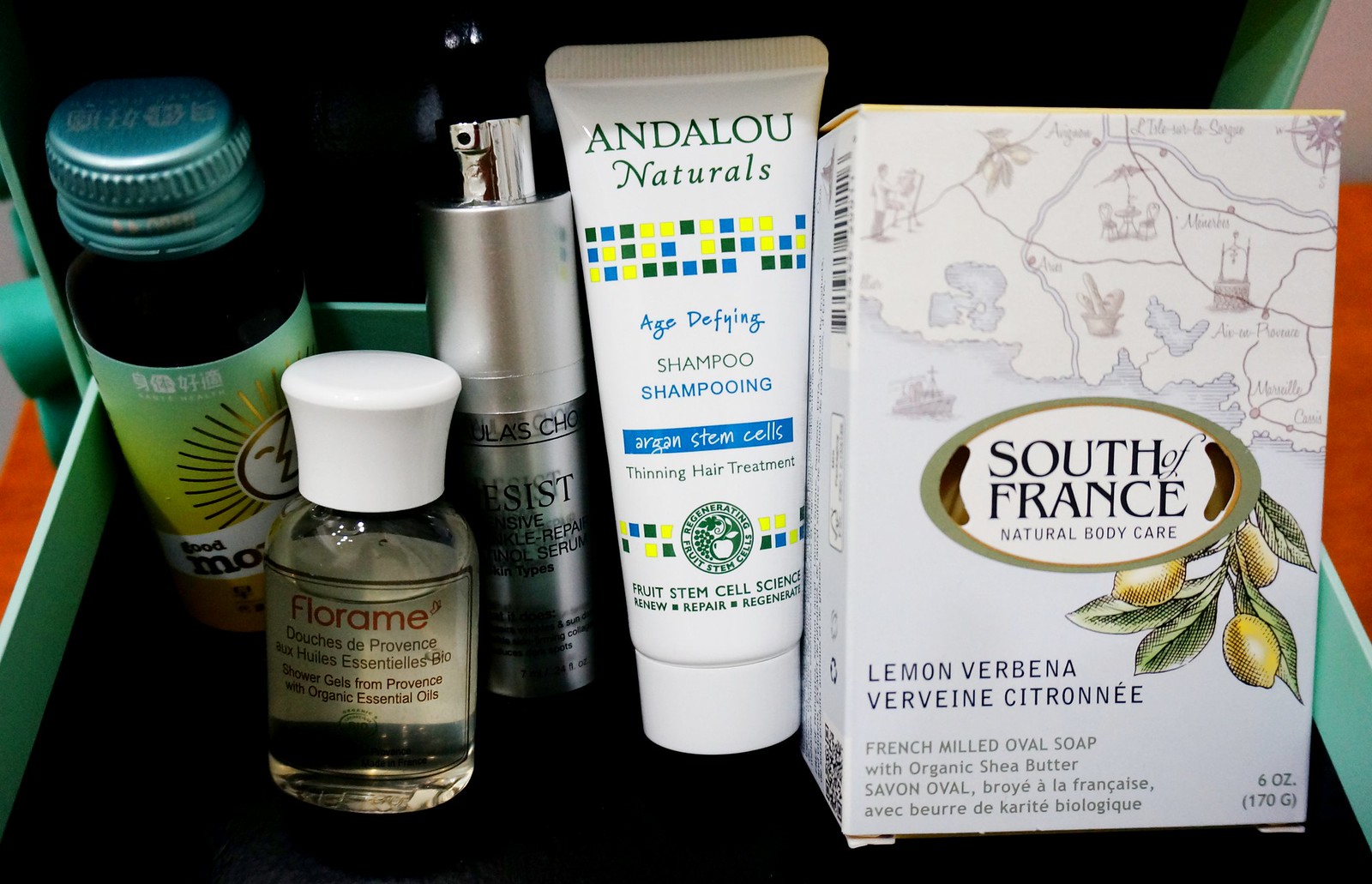The image showcases an assortment of toiletries neatly arranged within a green square box. Among the items is a large, oval soap encased in a white box, adorned with an illustration of a tree bearing lemons, suggesting a natural body care product with a lemon essence. Adjacent to it is a bottle of "Age-Defying Shampoo" by Andalou Naturals. This shampoo, intended for treating thinning hair, features the benefits of argan stem cells and comes in a white container accented with blue and yellow lettering.

The collection also includes a medium-sized, gray pump bottle with black lettering, though its precise contents are obscured by a shadow. A smaller, transparent container labeled "Florami" holds essential oil and is topped with a white cap.

Lastly, there is a container with a screw cap, displaying an image of a sun and some Asian script; the specific nature of this item remains unclear due to the limited visibility of the label. The entire set rests inside a green box, which appears to have a red accent on either side and possibly a matching green lid.